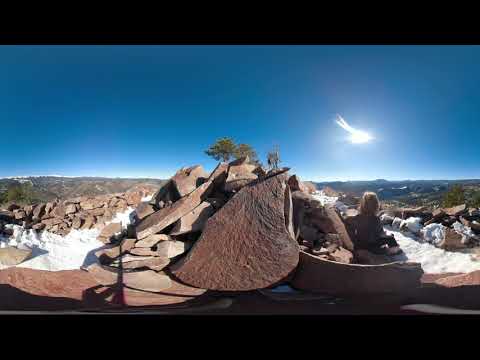This photograph captures an expansive and unique landscape filled with brown, flat rock formations stacked like panels, resembling steps that create a hill or elevated ground. Amidst the rocky terrain, patches of snow are scattered across the ground, adding a striking contrast to the earth-toned scene. Positioned on one of these rock formations, slightly to the right, a person, possibly a woman, sits contemplatively, adding a human element to the rugged natural setting.

The image reveals a vast panoramic view with distant mountains and multiple green trees standing out against the vibrant scenery. Above the landscape, the sky is a mesmerizing gradient of dark to bright blue, subtly touched by a bright white glare or light source that occupies the middle to the right top corner, vaguely resembling a bird-like shape.

The photograph stands out with its high brightness and distinct dark patches, framed by black borders at the top and bottom. The overall scene is both serene and thought-provoking, merging the raw beauty of nature with a contemplative moment.